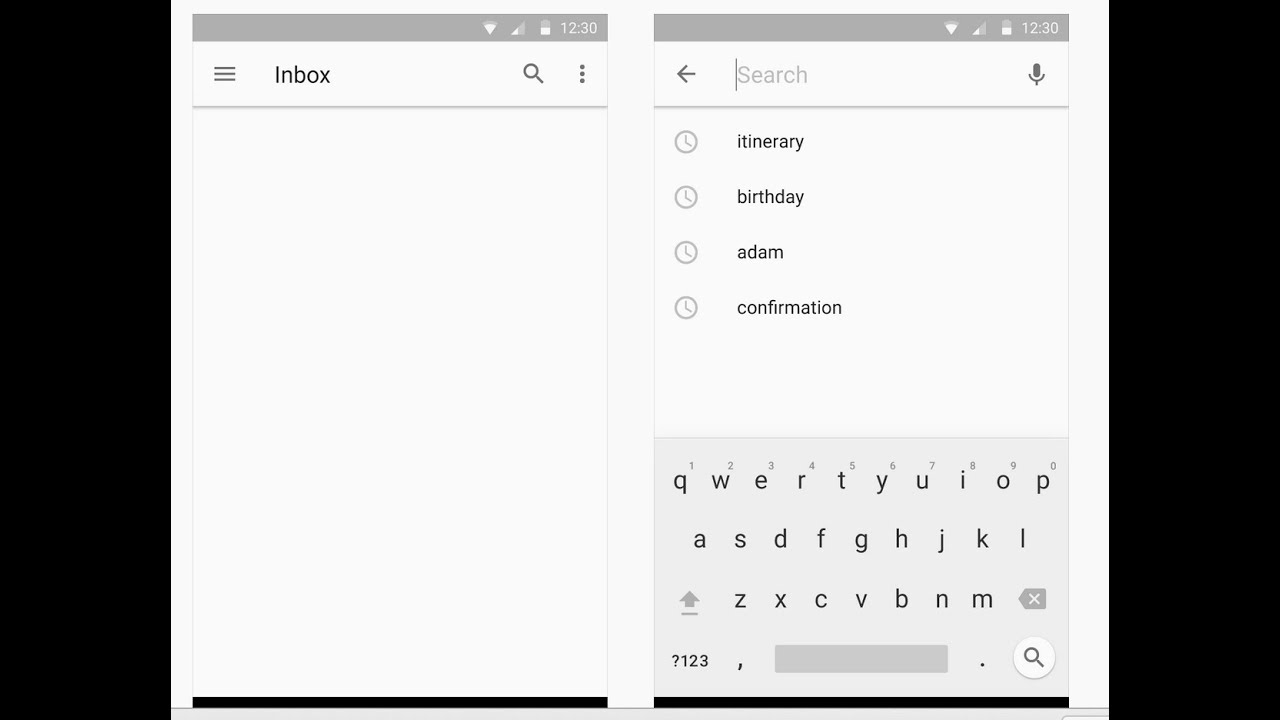The image features a pair of side-by-side screenshots. The left screenshot prominently displays an empty "Inbox" at the top, with a completely blank space below it. The right screenshot, labeled "Search," shows a blinking cursor in a search bar at the top. Underneath the search bar, a list of previously searched items is visible, including "Itinerary," "Birthday," "Adam," and "Confirmation." A virtual keyboard is displayed at the bottom of the screen, suggesting that the user is in the process of typing or searching for something.